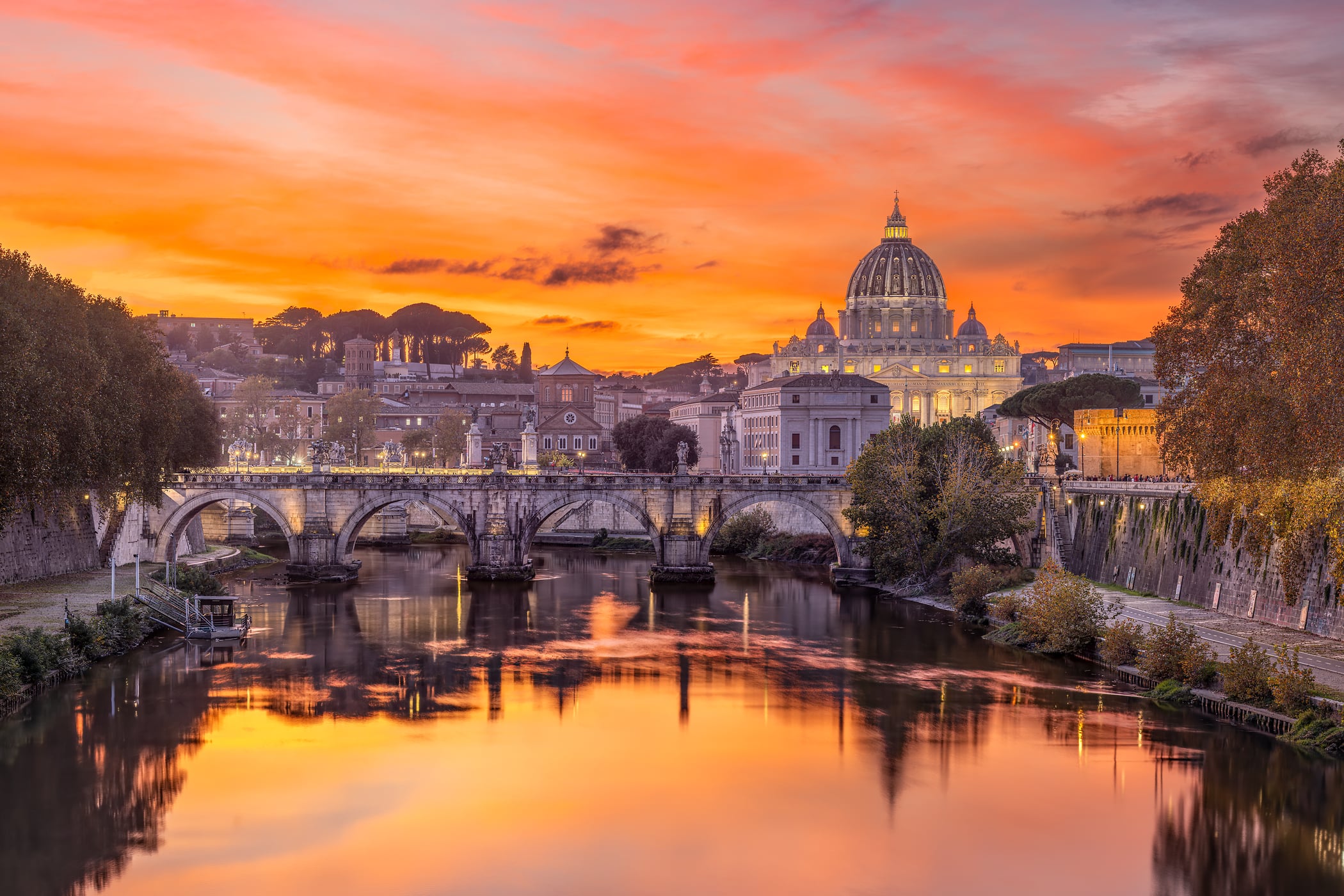This breathtaking landscape image showcases an exquisite depiction of old European architecture, centered around a beautifully illuminated temple or church with a dominant dome, reminiscent of a capitol building. The setting is during a vivid sunset, with a mesmerizing sky painted in shades of orange, yellow, pink, and light blue-violet, all of which are reflected strikingly in the tranquil waterway. The canal or river starts at the forefront of the image, extending away from the viewer, and is adorned with streetlights and lined by lush trees and shrubs. A prominent bridge with four grand arches spans the water from left to right, enhancing the majestic aura of the scene. The backdrop features additional buildings, indicating a residential and professional area, while the serene waterway flows continuously through this picturesque townscape.